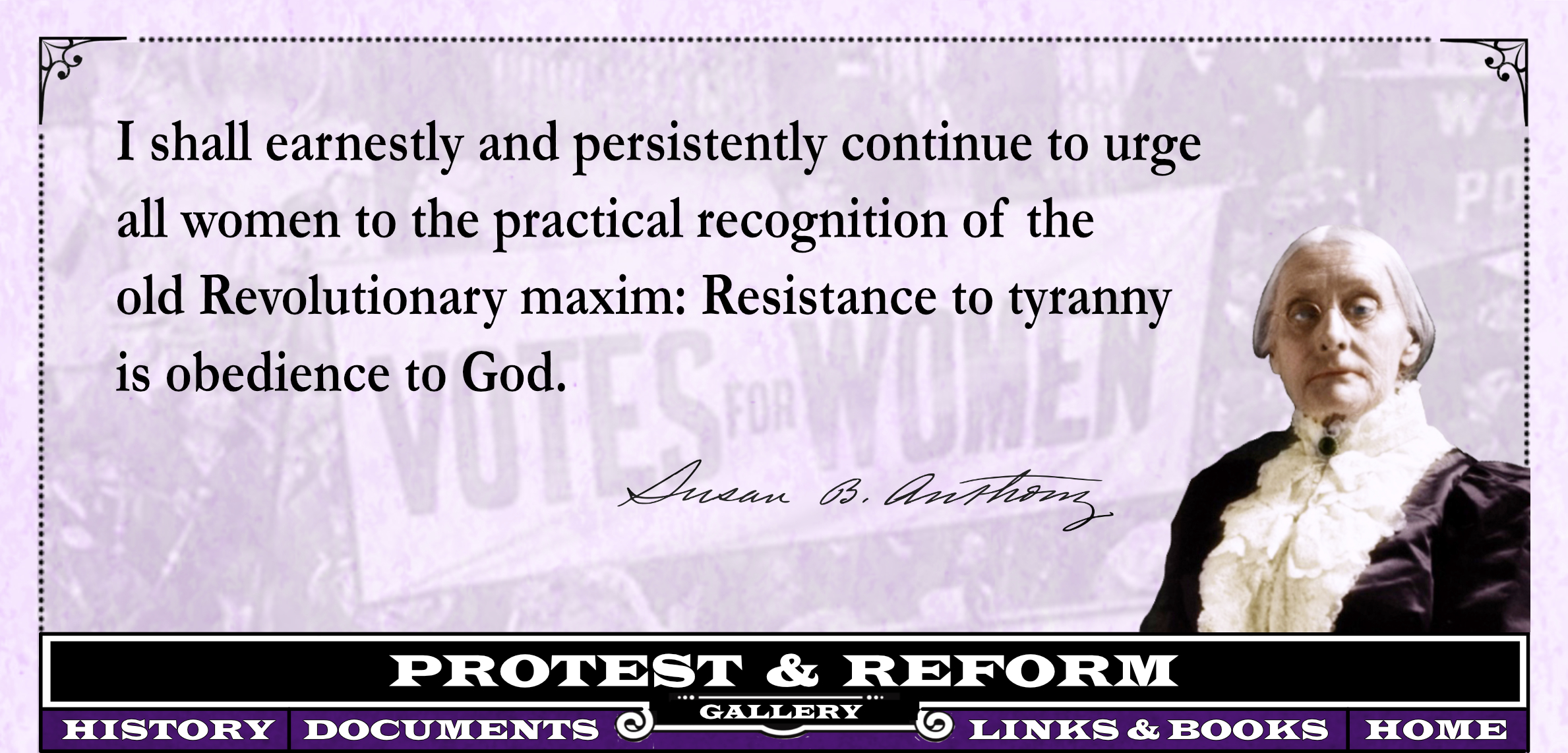The image resembles a rectangular landscape advertisement or digital flyer, styled like a vintage currency bill with a purple-tinted background. Dominating the design, a bold, black text quote by Susan B. Anthony reads: "I shall earnestly and persistently continue to urge all women to the practical recognition of the old revolutionary maxim: resistance to tyranny is obedience to God." This quote is left-justified and spans four lines. Beneath it on the right, her name appears elegantly in cursive. In the bottom right, there is an older woman, likely Susan B. Anthony herself, with white hair pulled back, high on her forehead, and wearing a severe expression. She sports a white, ornate, and frilly top that extends up to her neck, contrasting with the dark purple fabric on her arms and chest. The background features a faded sign reading "VOTES FOR WOMEN," indicative of a historical protest scene. At the bottom, a black bar in white text states "protest & reform," and below that, a purple bar with white text provides navigation options labeled "HISTORY," "DOCUMENTS," "LINKS & BOOKS," and "HOME."